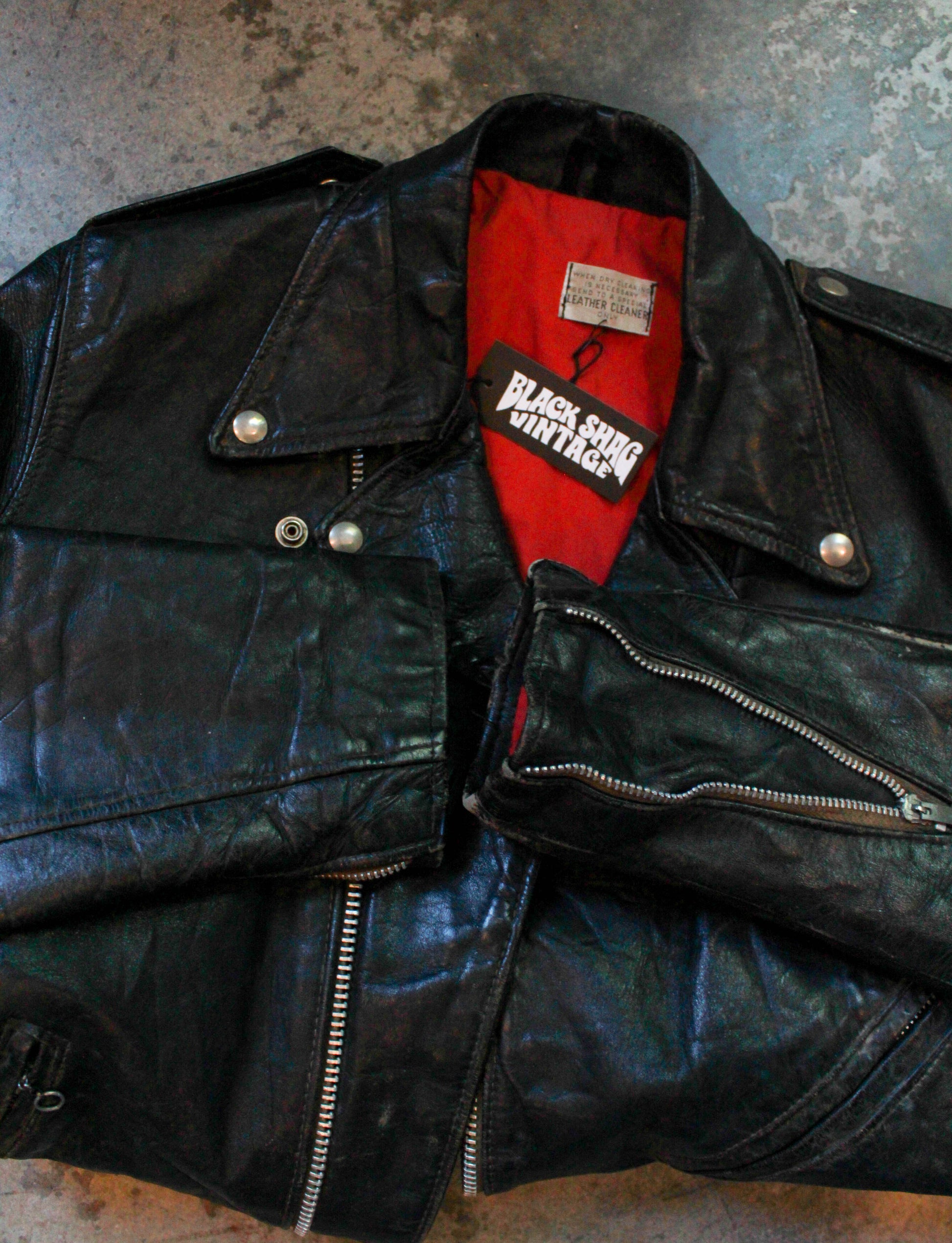The image depicts a well-worn black leather jacket with a vintage aesthetic lying on a concrete floor. The jacket has a shiny, smooth, and wrinkled texture, emphasizing its aged character. It is positioned with its arms folded over the front and the bottom folded underneath. Notably, a sleeve zipper runs from the wrist up a few inches, allowing adjustments for different wrist sizes with additional material between the zippers. The jacket features a zipper on the left side, a zippered pocket on the right, and silver buttons on the collar securing it to the chest. Silver shoulder straps, which could theoretically hold a sergeant patch but are not standard military issue, add to its design. The inside lining is a striking red, with a prominent tag that reads "Black Shag Vintage" in white. This tag is attached near an older one indicating leather cleaner instructions. The aged concrete floor adds to the overall retro vibe of the scene.